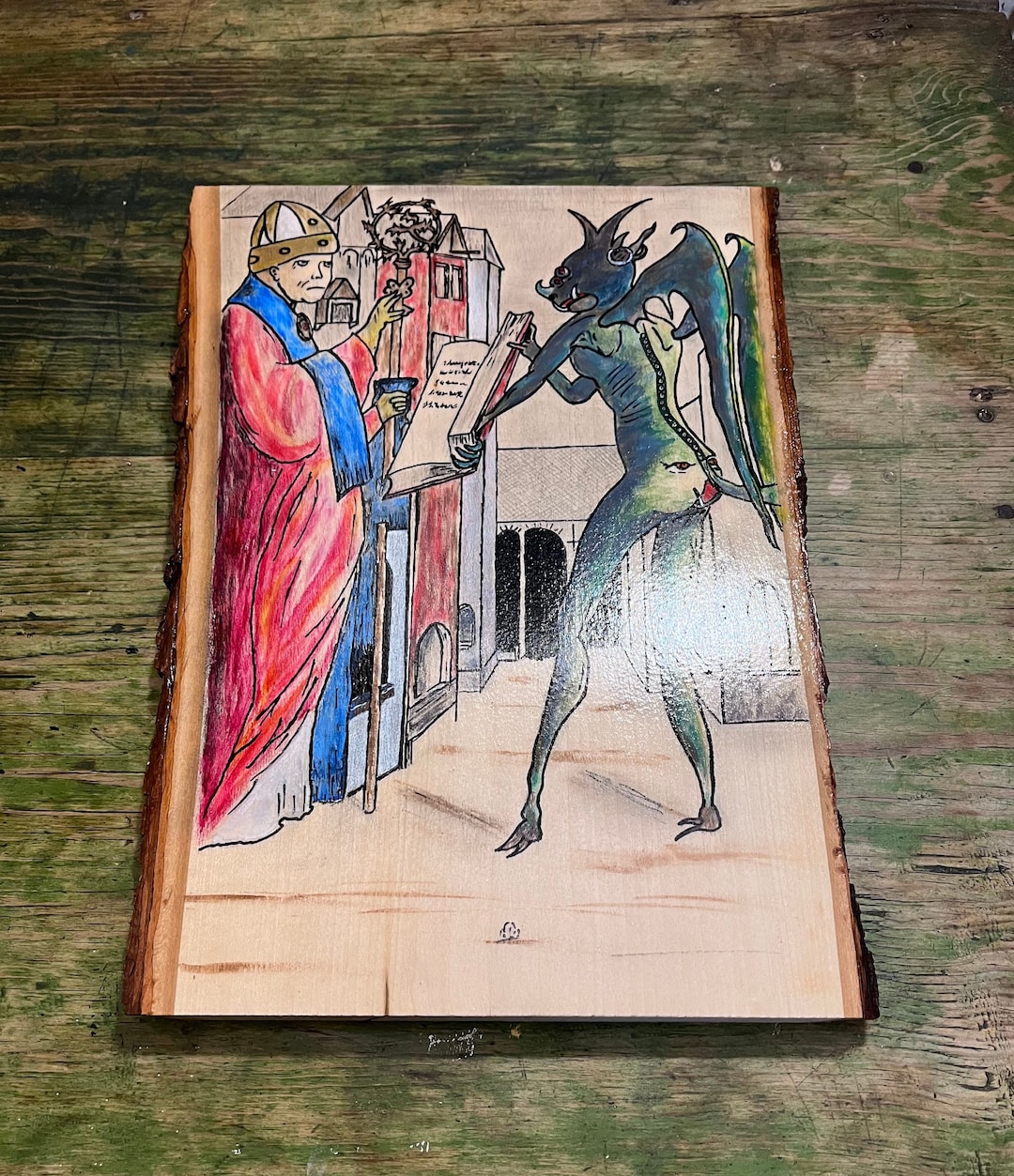The image depicts an intricately painted scene on a vertical, flat-cut piece of wood with dark bark lining the left and right edges. The wood itself has a glossy finish and serves as a canvas for the art. On the left side of the painting stands a religious figure, possibly a priest or Pope, dressed in a pink robe and a blue sash, with a gold and white hat or helmet. He holds a chalice or staff in his left hand and reaches out with his other hand.

To the right of the priest stands a green devil-like creature with dark green wings, a lizard-like face with red eyes, and horns protruding from its head, including one for a nose. The creature has two hooves and appears to have a zipper on its back, suggesting a mixture of human and fantastical elements. It holds an open book towards the priest, revealing pages with black writing.

The background features various buildings, predominantly red, light blue, and brown, standing against a cream-colored sky. These structures are nearly as tall as the figures themselves, indicating a surreal scale. The entire painted scene resides on a green and beige wooden table, complementing the natural tones of the wood canvas.